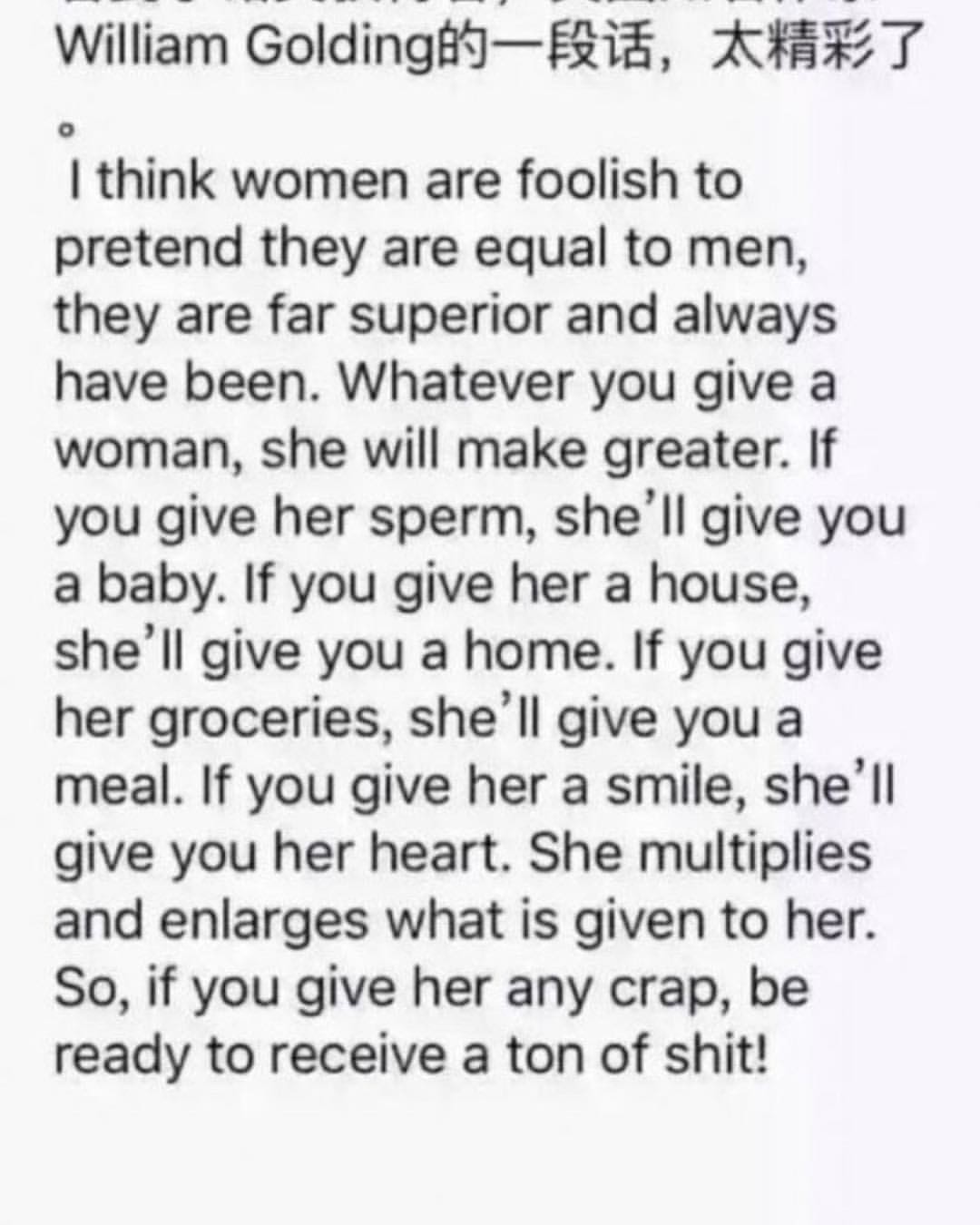The image is a photograph of a white page with black text. At the very top, it reads "William Golding" followed by some Asian characters, possibly Chinese or Japanese. Below this, there is a significant gap before the main body of text. The text, presented in a single black paragraph, reads: "I think women are foolish to pretend they are equal to men; they are far superior and always have been. Whatever you give a woman, she will make greater. If you give her sperm, she'll give you a baby. If you give her a house, she'll give you a home. If you give her groceries, she'll give you a meal. If you give her a smile, she'll give you her heart. She multiplies and enlarges what is given to her. So, if you give her any crap, be ready to receive a ton of shit!" The overall image has a simple and clean layout with just the white background and black text, emphasizing the message without any additional colors or imagery.